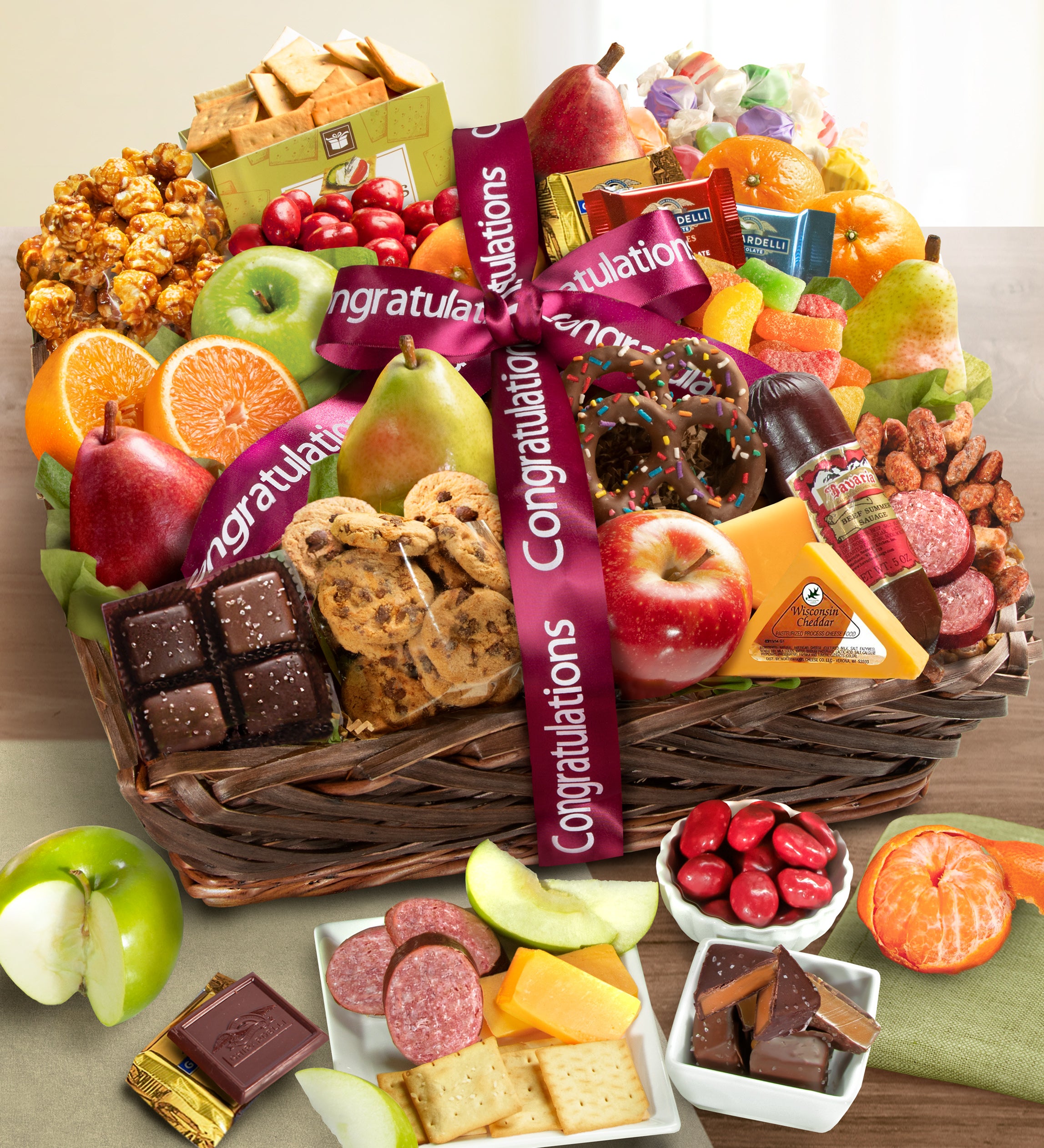In this photograph, a woven dark-brown gift basket adorned with a maroon ribbon that reads "congratulations" is the focal point. The basket contains a vibrant assortment of fruits, snacks, and desserts. Prominently displayed in the basket are different types of fruits including green apples, red apples, a green pear, a red pear, cherry tomatoes, an orange cut in halves, and a half-peeled tangerine or orange resting on a green napkin. There is also an array of sweets and snacks, such as Ghirardelli chocolate, chocolate chip cookies, chocolate-covered candy, chocolate-covered pretzels with colored sprinkles, caramel corn, and blocks of cheese. 

On the table beneath the basket, which is set against a plain white wall, there are several plates and serving dishes. One white, square serving dish holds sausage slices, crackers, sliced apples, and cheese. Another square dish features some type of chocolate pastry, while a round dish contains what looks like Boston peanuts. The entire composition is meticulously arranged on a wooden table, which emphasizes the diverse and colorful contents of the gift basket.